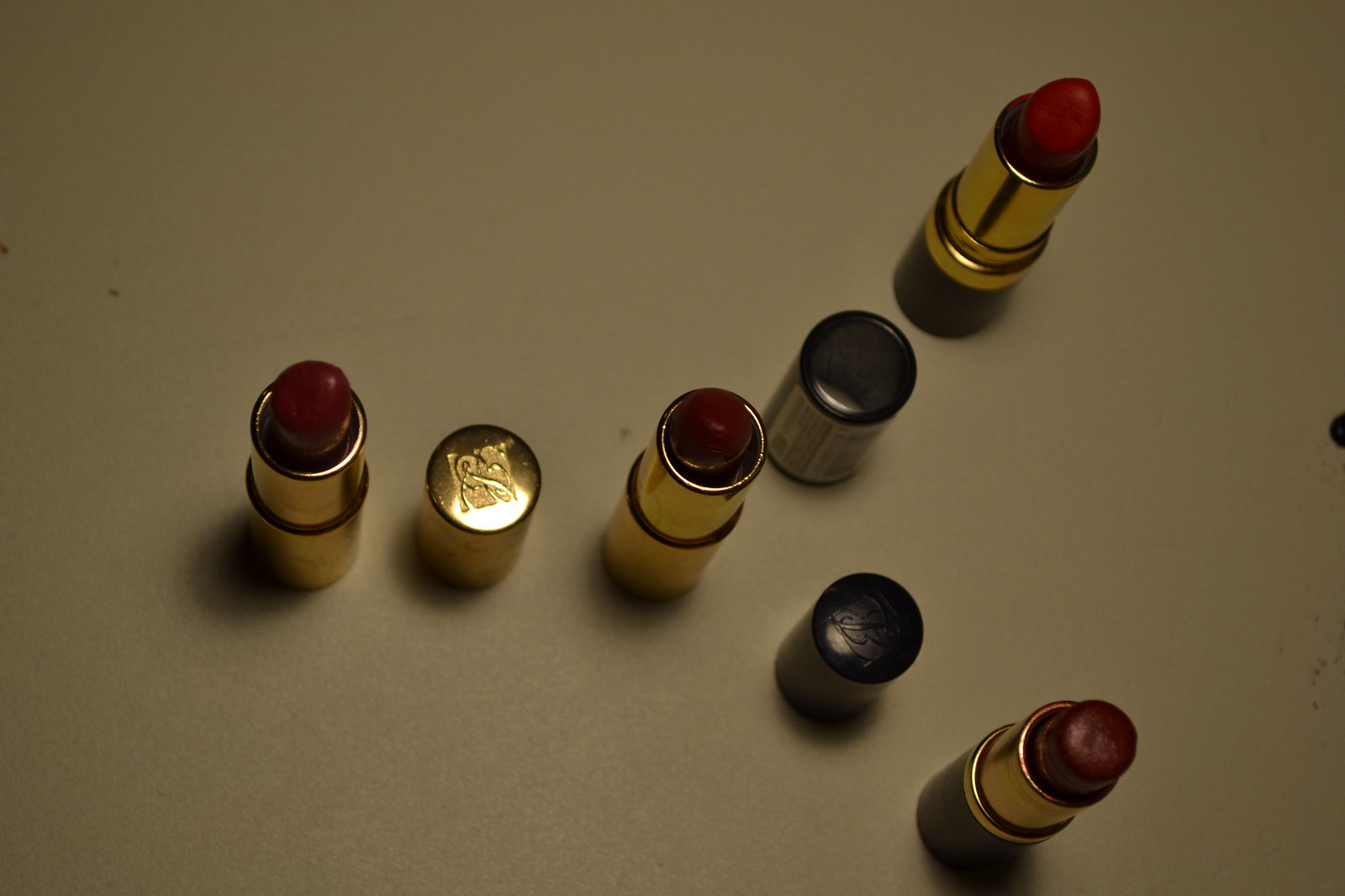This indoor, slightly out-of-focus photograph captures a collection of four used lipsticks arranged on a white surface, taken from an overhead angle. The lipsticks are meticulously positioned to form a sideways "Y," with the stem extending to the left and the open end to the right. The background features a light green and light tan hue, adding to the overall dim and dark ambiance of the image. 

Each lipstick container features a golden cylinder, although the caps vary in color. Starting from the left, the first lipstick is a deep red shade, with its cap—adorned with some scroll work but no readable text—placed adjacent to it. Next to it, another identical golden tube is positioned, accompanied by two black caps slightly above and below. One of the black caps appears to have a tag or a worn label, possibly a UPC code, and might display a faint "B" marking on one. Moving to the top right, another lipstick in a similar golden tube but with a black bottom is visible. The fourth lipstick, located at the lower right, mirrors the design of the third with its black bottom and golden tube, containing the same dark red shade. 

Notably, the lipstick at the lower right corner is the brightest shade of red among them. Despite the well-structured arrangement, a light glare is visible, possibly from the camera, but no text or additional objects are visible within the frame. In the far right corner, a hint of something dark, possibly a dog or part of another object, is barely discernible. The careful arrangement and varied details of the lipsticks create a visually engaging yet subtly lit composition.